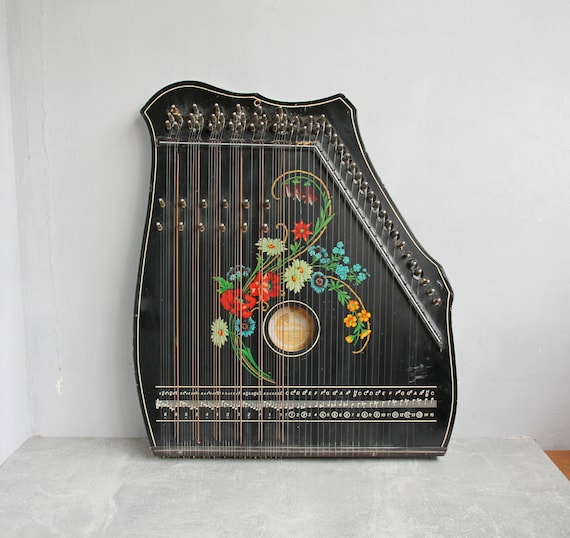The photograph captures a black autoharp prominently centered on a white table against a white wall with a wood floor visible beneath. The autoharp’s body is adorned with an intricate, colorful floral design that includes white daisies, red, yellow, orange, blue, and deep dark purple flowers. This floral pattern intricately curves around the central acoustic hole in a reverse S shape, creating a bouquet-like effect. The strings, numerous and silver, are meticulously arranged, with the tuning knobs located at the top of the instrument. The instrument's ornate detailing and the delicate balance of its components highlight its complex and decorative craftsmanship.